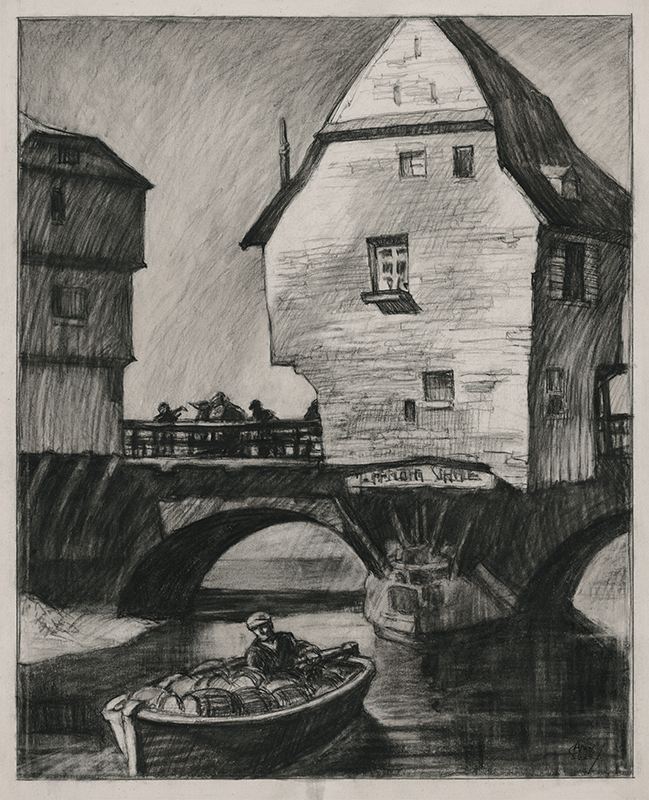This is a detailed sketch rendered in black and white, with the medium appearing to be a black pencil on light gray paper, providing an old-world charm. Central to the composition is a stone arched bridge, showcasing two prominent arches under which a river flows. The bridge itself is adorned with architectural elements: on its columns or posts, two distinct buildings stand out. 

To the right, there's a stone-faced house with a triangular roof, featuring at least two levels. Its roof is interestingly detailed, transitioning into a slanted section with a chimney on one side. The windows have a lattice design, adding to the intricate beauty of the structure. On the left side of the bridge, you see another house, possibly three stories tall, distinguished by its steep, fast roof.

People populate the scene—some strolling across the bridge, others peering over the sides into the river below. The river is alive with activity, notably featuring a small rowboat loaded with cargo. The man rowing appears to be transporting goods, adding a narrative element to the tranquil scene. The water reflects the bridge and sky, with skillful shading effects suggesting reflections. The overall mood is nostalgic, evoking a time before modern inventions, enriched by the careful detailing of the architectural features and human activities.